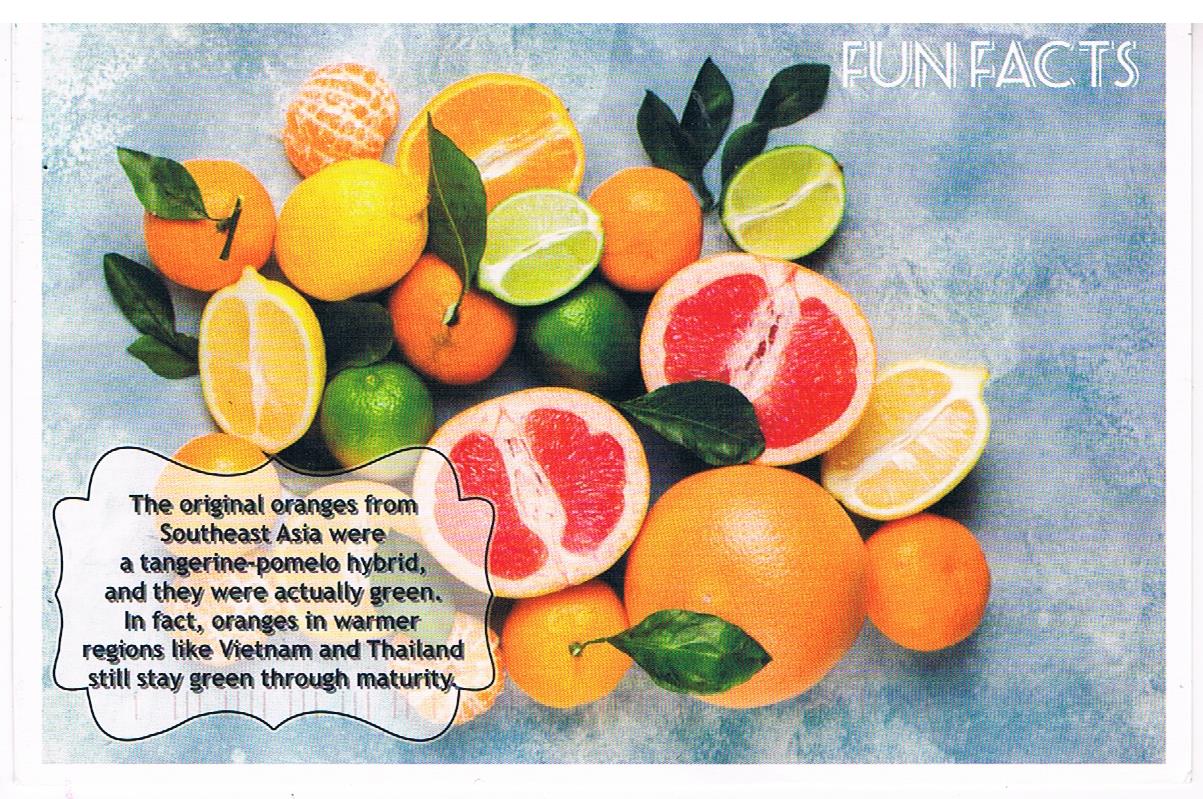This color photograph features a vibrant assortment of citrus fruits displayed against a sponged blue and white background. In the upper right-hand corner, the phrase "FUN FACTS" is prominently displayed in white capital letters. The fruits are artfully arranged, stretching from the upper left to the lower right of the image. There is a variety of oranges, lemons, limes, and grapefruits, with many cut in half to reveal their juicy interiors, while others remain whole. Some fruits even retain their green leaves and stems for added freshness. Among the fruits is a peeled half-orange, a lemon and lime cut in halves, and a grapefruit cut in half, all positioned to face outward. In the bottom left corner, an irregularly shaped white box contains a fascinating fact in black writing: "The original oranges from Southeast Asia were a tangerine-pomelo hybrid, and they were actually green. In fact, oranges in warmer regions like Vietnam and Thailand still stay green throughout maturity."